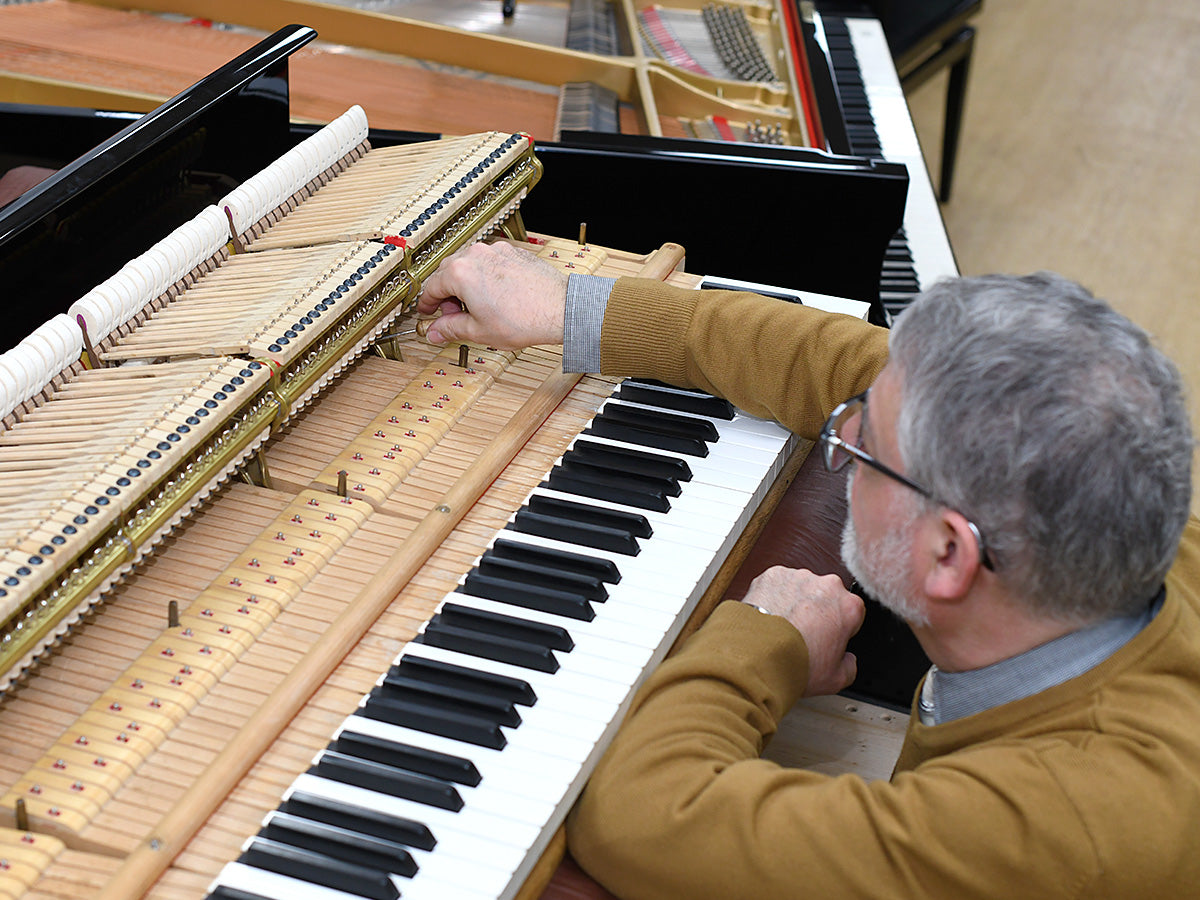In this detailed image, a man is meticulously working on a piano, its top lid propped open to reveal the intricate wooden mechanisms inside. The piano's key set, consisting of elongated white keys interspersed with shorter black ones, is clearly visible. The man, wearing a yellow sweater over a gray shirt, sports glasses and has gray hair, indicative of his meticulous nature. His attention is focused, using a small screwdriver with a wooden handle to adjust components between the layers of wooden mechanisms housed within the piano. The detailed mechanisms, mirroring the piano keys in form but constructed from wood, are arranged in two distinct levels. Behind him, another piano, part of a wooden floor, and a portion of a black stool can be seen, adding context to the environment. The man's careful work captures a moment of focused craftsmanship in maintaining the musical instrument.